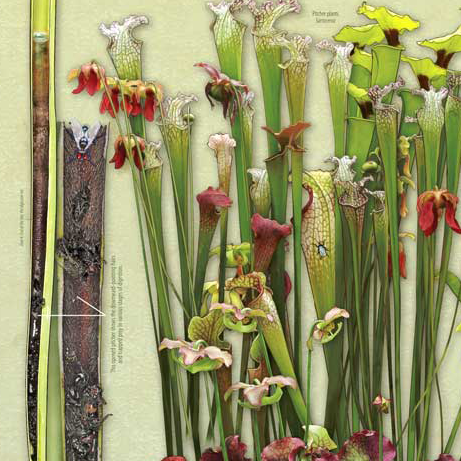The image depicts a page from a book featuring a detailed botanical illustration. The artwork showcases a variety of flowering plants characterized by their elongated green stems. These stems, however, exhibit a yellowish and somewhat frail appearance. Atop each stem, colorful flower petals are prominently displayed, with hues ranging from vibrant reds and purples to delicate whites and yellows. Some flowers appear wilted and are situated lower on the stems, while the fresher, more vibrant blooms are positioned higher up. On the left side of the page, there is annotated text or markings, and two lines extend towards a dark gray, stick-like object, possibly indicating some form of botanical notation or reference.